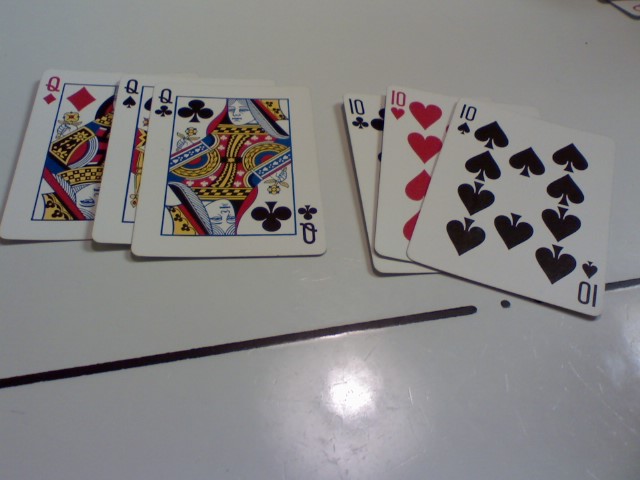The photograph captures a meticulously arranged set of playing cards placed on a flat, white, glossy, and reflective surface. The image is rectangular, with the longer sides at the top and bottom and shorter sides on the left and right. Dominating the bottom edge and the top right corner are prominent black lines, and the surface bears multiple scratches, evidencing previous use. 

In the bottom center of the image, a round, white light is reflected, likely emanating from a ceiling fixture. Two distinct piles of cards are neatly stacked, each containing three cards. The left pile features queens: at the bottom is a red Queen of Diamonds, followed by a black Queen of Spades, topped with a black Queen of Clubs. The right pile showcases tens: beginning with a black Ten of Clubs at the bottom, then a red Ten of Hearts, and capped with a black Ten of Spades.

The arrangement and details of the cards are clearly visible, making the image both visually interesting and rich with texture.